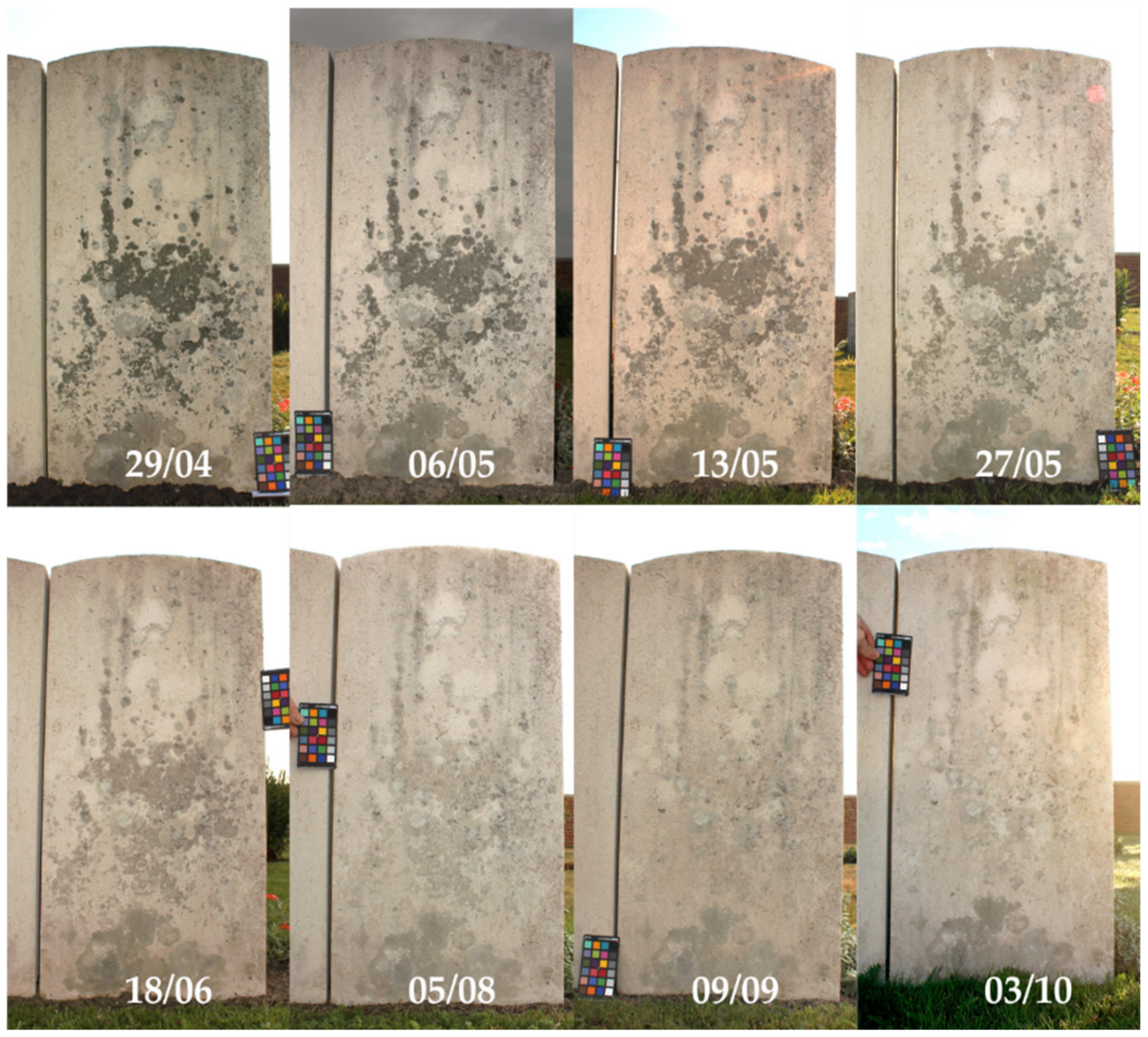This image depicts a series of eight granite slabs arranged in a grid pattern, resembling tombstones but without any engravings. Each granite slab features what appears to be a rectangular color palette with multicolored squares beside it. Beneath each slab, there is a series of dates inscribed in a "dd/mm" format, ranging from April 29th to October 3rd. The dates sequentially progress from the top left to the bottom right as follows: 29/04, 06/05, 13/05, 27/05, 18/06, 05/08, 09/09, and 03/10. The granite slabs are primarily whitish-gray in color and initially have green splotches or dirt marks on them. However, as the dates progress, these splotches become lighter and less noticeable, suggesting a gradual cleaning or weathering process. Each image within the series includes the presence of a person who might be holding or leaning a colorful piece of paper against the slabs.